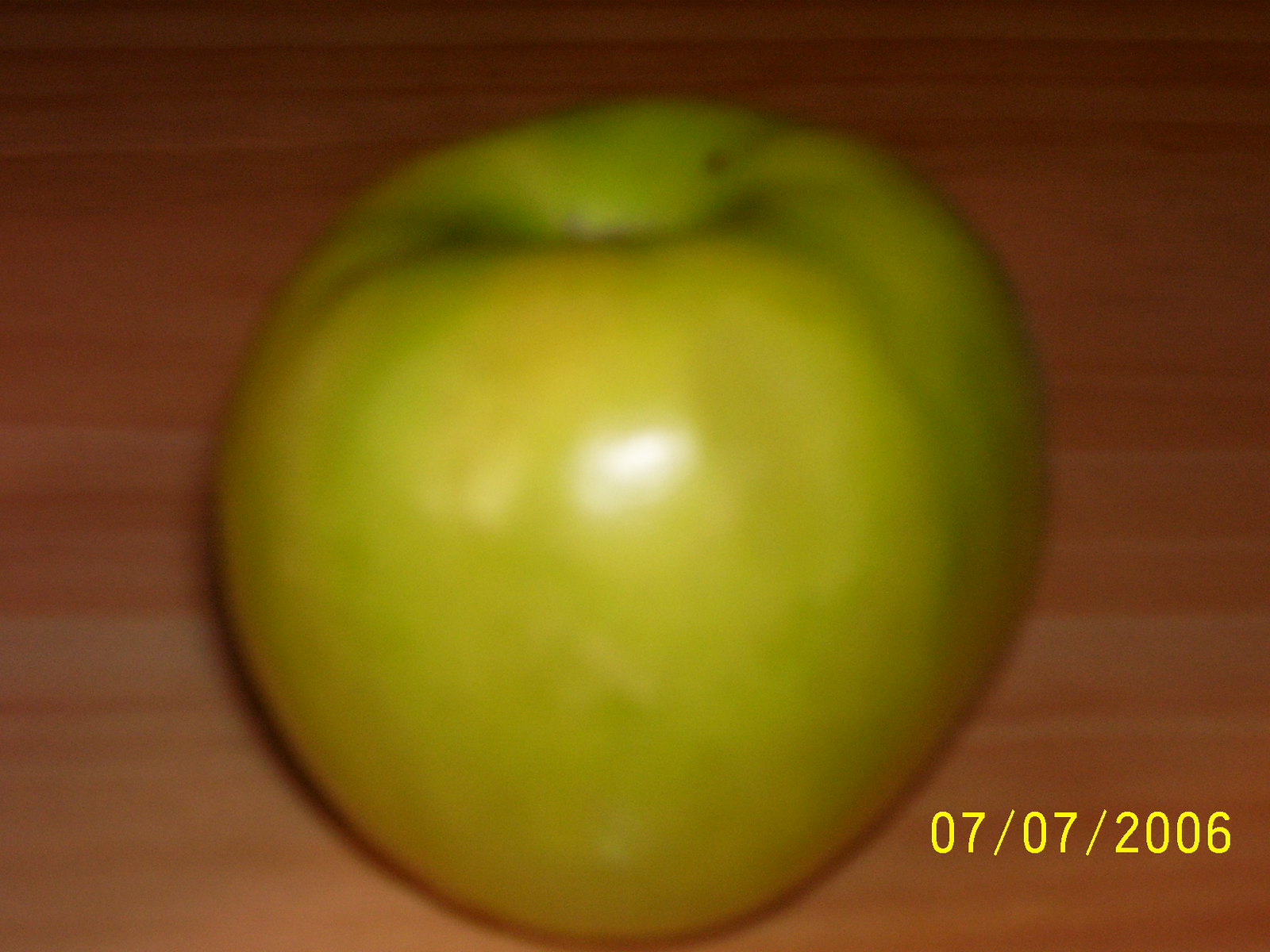A close-up, slightly blurry photograph captures a classic green apple resting on a wooden surface. The apple exhibits various shades of green interspersed with hints of yellow, and towards the top, near where the stem would be, a subtle reddish tint. There's a small black dot, larger than a pinhead but not overly significant, positioned at roughly one o'clock on the apple. Light reflects off its smooth skin, providing a glossy sheen. On the lower right-hand corner of the photograph, large yellow text indicates it was taken on 07-07-2006. Shadows cast predominantly on the left side of the apple suggest a light source from the right, with the deepest shadow pooling under the lower left-hand section of the fruit.